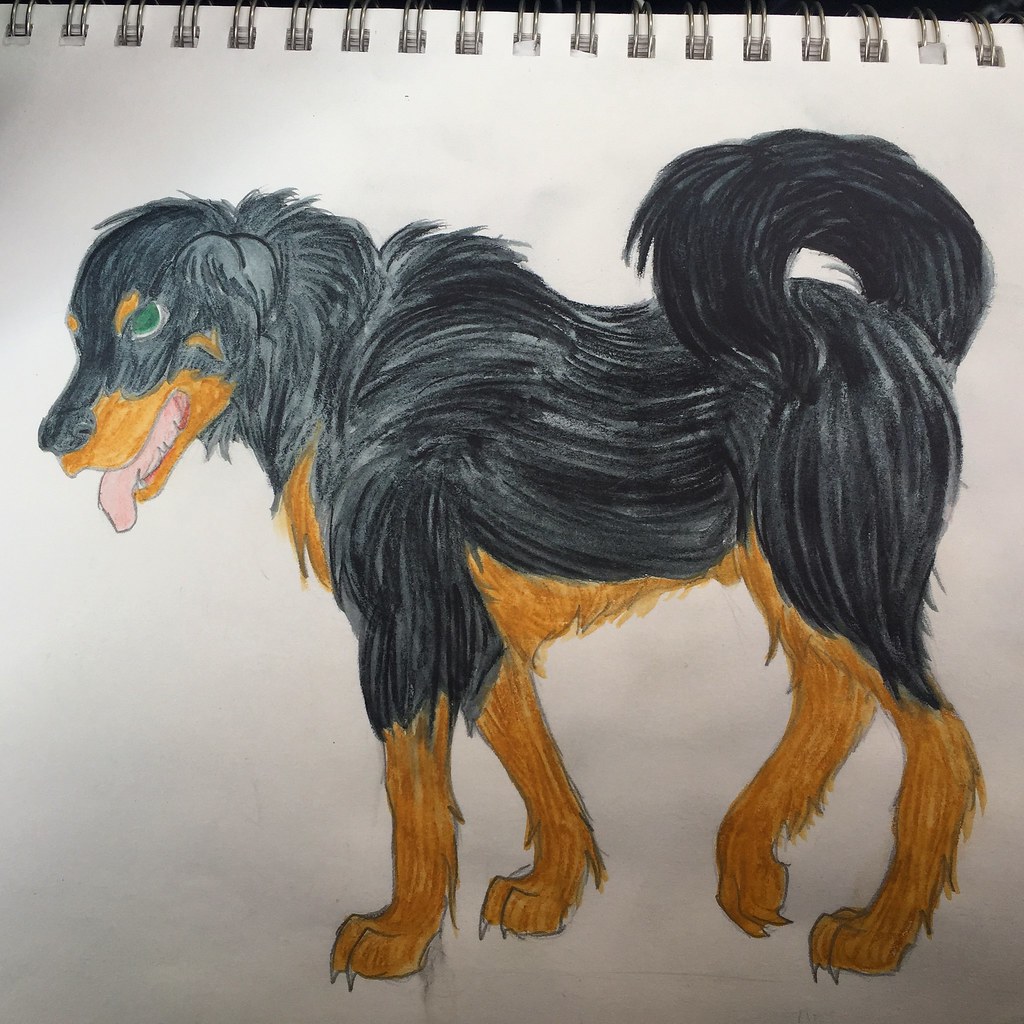This detailed drawing, rendered on a white spiral-bound art pad, showcases a meticulously illustrated dog with long fur. The dog, positioned centrally and facing left, is predominantly black along the back while its underbelly, legs, and areas around the mouth are a contrasting tan. The artist has expertly used black and brown crayon to bring depth to the dog's features, which include green eyes, a pink tongue hanging out in a panting expression, and detailed claws visible on each paw. The tail arches gracefully over the dog's back, adding to the lifelike depiction. The light and shadows within the white paper accentuate the careful attention to detail, enhancing the overall realism of the drawing.